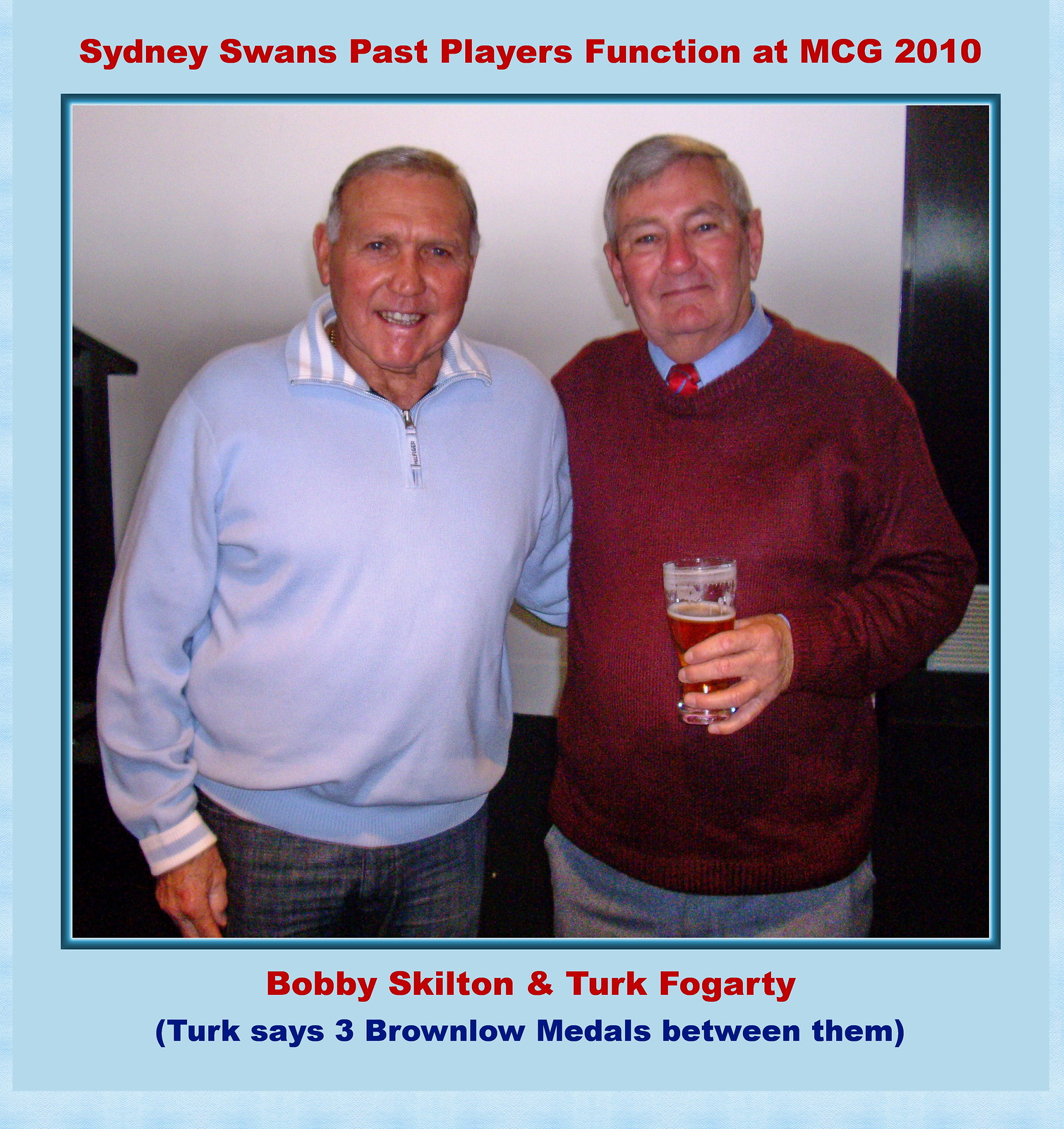The photograph depicts two older men with grey hair standing side by side, smiling in front of a white wall. The man on the left is dressed in a light blue pullover sweatshirt with a zipper and jeans. The man on the right is wearing a red sweater and a red tie underneath, and he is holding a glass of dark red beer in his left hand. Above them, red text reads, "Sidney Swann's Past Players Function at MCG 2010." Below the image, red text identifies the men as "Bobby Skilton and Turk Fogarty," and underneath this, blue text in parentheses notes, "Turk says three Brownlow medals between them." The image is framed by a blue border set against a light blue background.